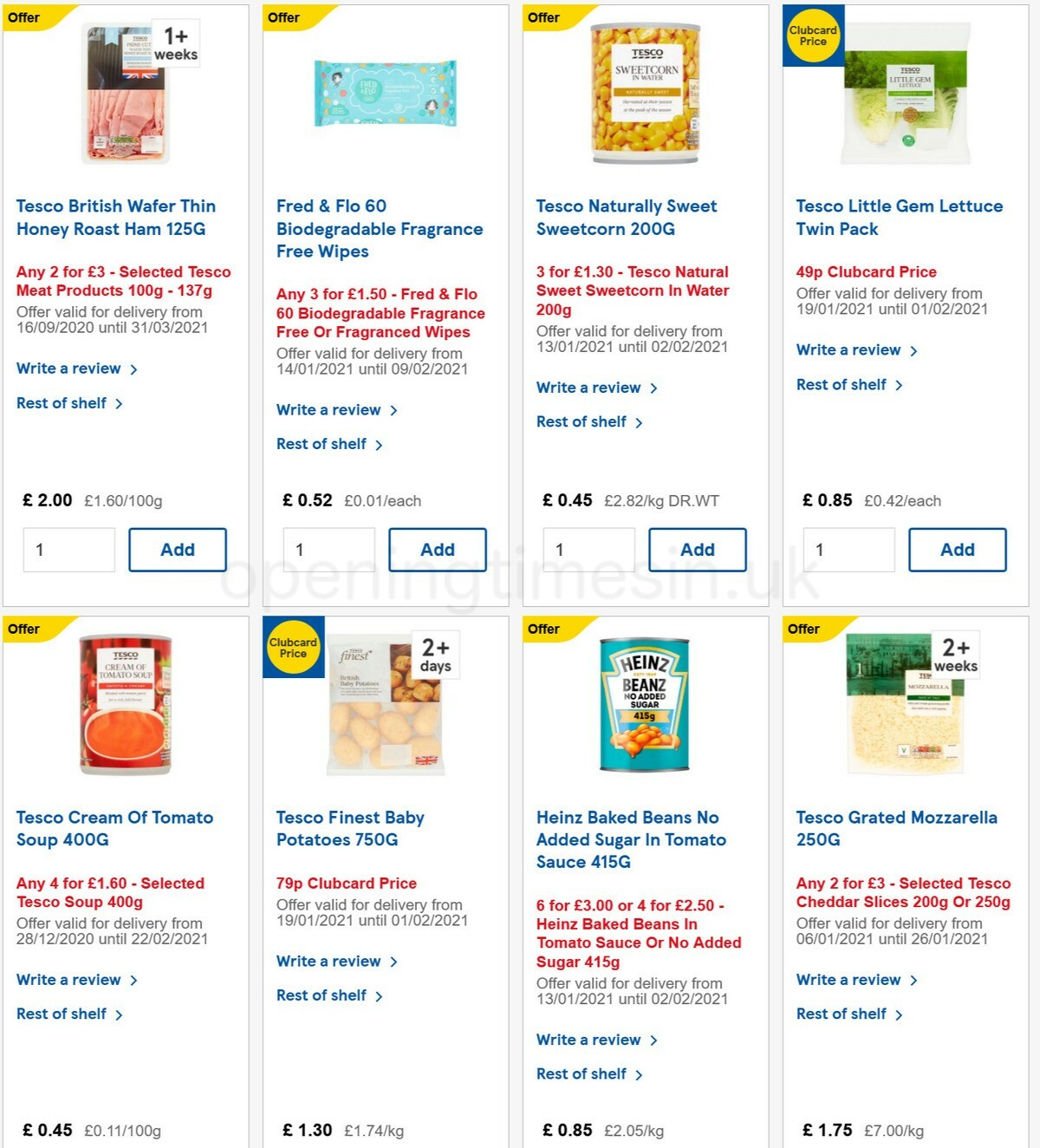The image showcases a Tesco supermarket webpage featuring eight different grocery items arranged in a grid layout, with four items in the upper row and four in the lower row. The first item on the upper left is Tesco British Wafer Thin Honey Roast Ham, which is available for delivery from 16-09-2020 until 31-03-2021 at a price of £2, accompanied by an 'Add' button. Moving to the right, the next product is Fred and Flo 60 biodegradable fragrance-free wipes. The third item is Tesco Naturally Sweet Sweet Corn, followed by Tesco Little Gem Lettuce Twin Pack on the far right of the top row. On the bottom row, starting from the left, the first item is Tesco Creamer Tomato Soup. Next to it is Tesco Finest Baby Potatoes, followed by Heinz Baked Beans with no added sugar in tomato sauce. The final item on the bottom right is Tesco Grated Mozzarella. Each product listing is complete with an image, product description, and functionality to add the item to a shopping cart.